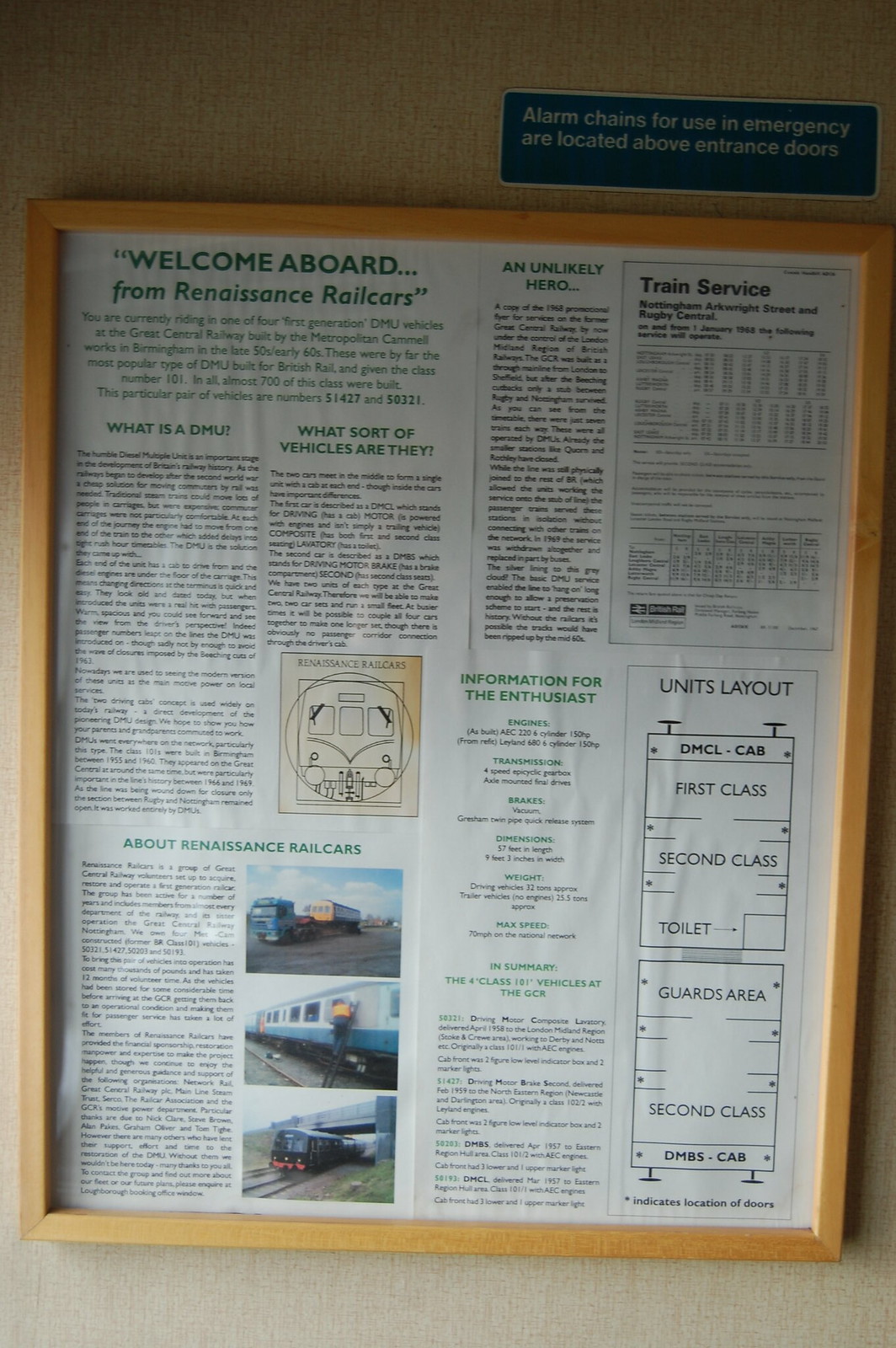Located on the neutral tan wall of a train, there's a detailed sign enclosed in a natural wooden frame. The sign, resembling a page from a newspaper with four columns, is titled "Welcome Aboard from Renaissance Rail Cars." Above the sign, there is a noticeable blue rectangular emergency sign with white outlines and white font, stating "wrong things for use in an emergency are located above entrance doors." The paper features various black fonts and some green-highlighted text, providing extensive information about the train services. Notably, within the right side column, there is a table typically used to display box arrangements. The sign also includes at least three pictures of the train, with the second column showcasing a drawing of the front of the train, and the bottom featuring photographs. Additionally, the bottom right side of the sign illustrates a diagram detailing the train's layout, including first-class and second-class seating, and toilet locations. This meticulously presented information offers a glimpse into the restored Renaissance Rail Cars and their services.